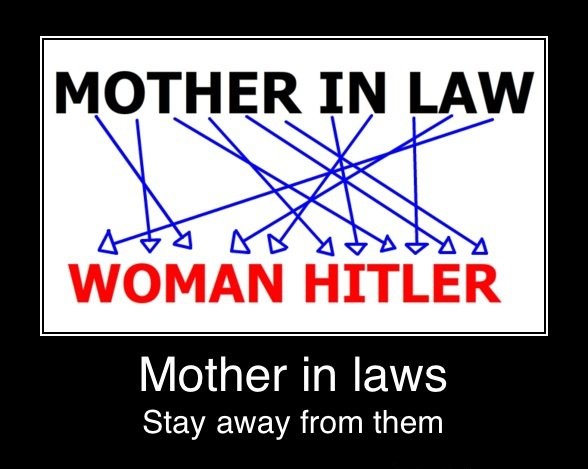The image resembles a slide from a presentation, featuring a plain black background with a central white box bordered with a double black and white border. The white box contains all-caps black text at the top that reads "MOTHER-IN-LAW" and red text at the bottom that reads "WOMAN HITLER." A series of overlapping and scattered blue arrows point downward from "MOTHER-IN-LAW" to "WOMAN HITLER," suggesting a transformation or unscrambling of the text. Below the white box, larger white text on the black background states "MOTHER-IN-LAW'S," followed by smaller white text underneath that says "stay away from them." The overall layout resembles a motivational meme, typically designed to circulate on social media, and the clarity of positioning suggests it could be part of a PowerPoint presentation.